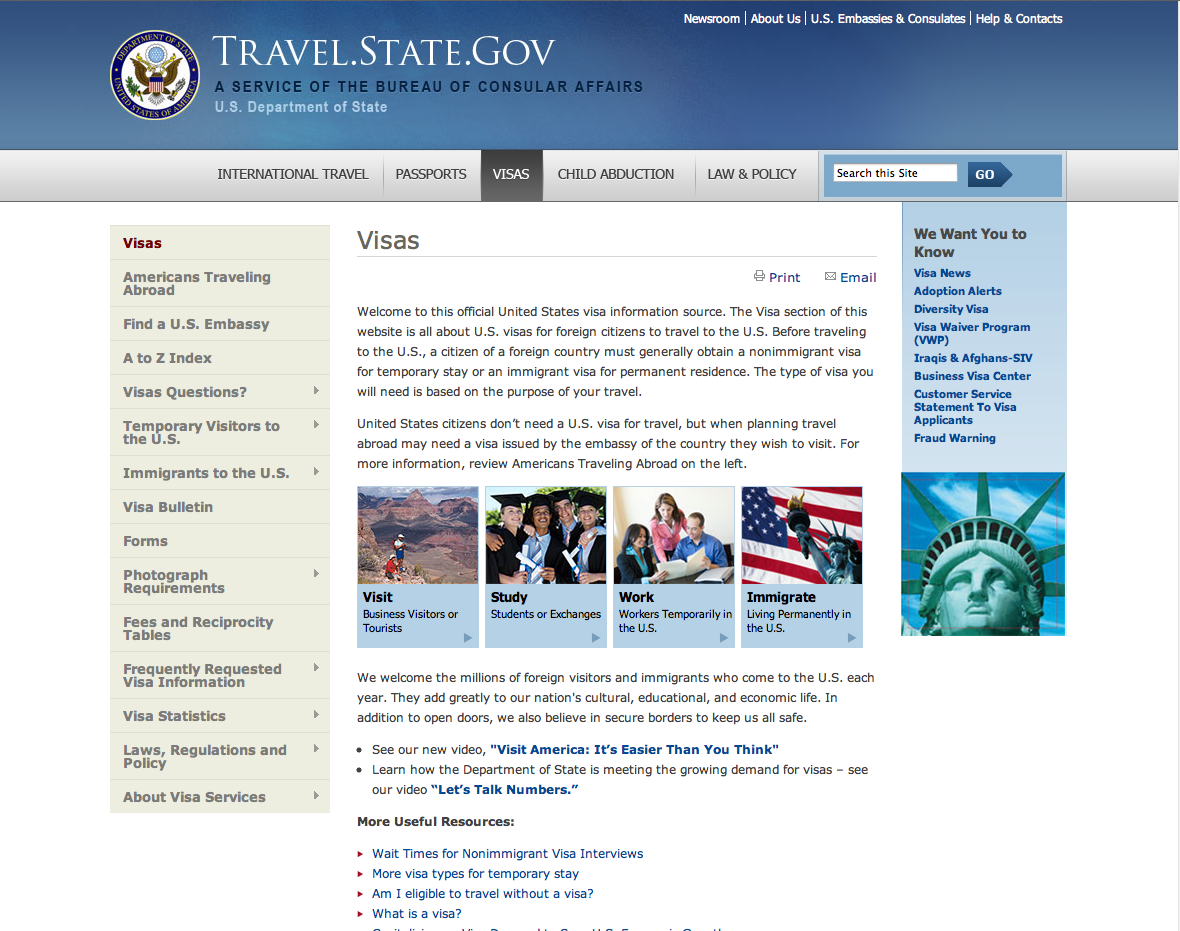The image depicts a webpage from travel.state.gov, a service provided by the Bureau of Consular Affairs of the U.S. Department of State. The page prominently features the emblem of the Department of State, showcasing an eagle with the American flag in a circular blue logo.

At the top of the webpage, there are several navigation filters including Newsroom, About Us, U.S. Embassies and Consulates, Help, and Contacts. The Visa section is currently selected. Other sections available are International Travel, Passports, Child Abduction, and Law and Policy.

The content of the Visa section welcomes visitors to the official United States visa information source. It provides detailed information about U.S. visas for foreign citizens who wish to travel to the United States. The text explains that foreign citizens need to obtain either a non-immigrant visa for temporary stays or an immigrant visa for permanent residence, depending on the purpose of their travel.

It is noted that U.S. citizens generally do not need a visa for traveling domestically, but may require a visa issued by the embassy of their destination country for international travel. There is a prompt directing readers to review the "Americans Traveling Abroad" section on the left for more information.

The page categorizes different types of visas into visit, study, work, and immigrant sections: 

- "Visit" for business visitors or tourists.
- "Study" for students or exchange visitors.
- "Work" for temporary workers in the U.S.
- "Immigrant" for those living permanently in the U.S.

Additional resources and a section titled "Things They Want You to Know" are also present. The page includes a visually striking image of the Statue of Liberty, highlighting its iconic green color and expressive face.